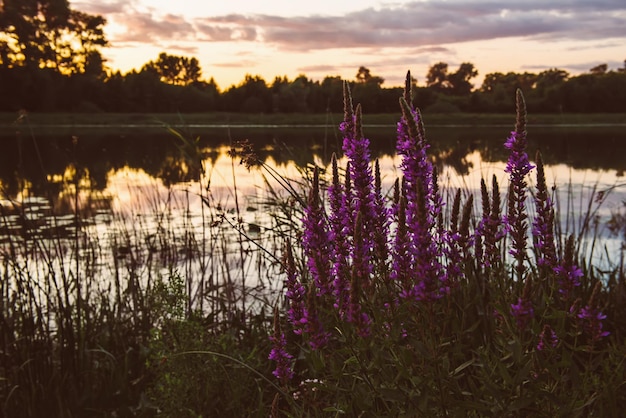This landscape photograph, taken during either sunrise or sunset, captures a serene moment by a still body of water, possibly a pond or a lake. The scene features a golden-yellow sun positioned in the upper left, casting an ethereal glow and causing dramatic reflections on the water's glassy surface. Surrounding the sun, gray clouds loom in the sky, adding depth to the scene. Along the horizon, a line of silhouetted trees stands against the sunlight, extending their reflections into the calm water below. 

The foreground is richly detailed with patches of tall grass and clusters of purple wildflowers to the right, characterized by their spiky, stalk-like appearance. Their vibrant color pops against the otherwise subtle and dark hues of the image. In the water near the shore, lily pads float serenely, further enhancing the tranquility of the scene. Despite the filter-like quality giving the photograph an old-school appearance, the image remains sharp, allowing for appreciation of the reflective stillness and the picturesque wildflowers that frame this peaceful moment beautifully.